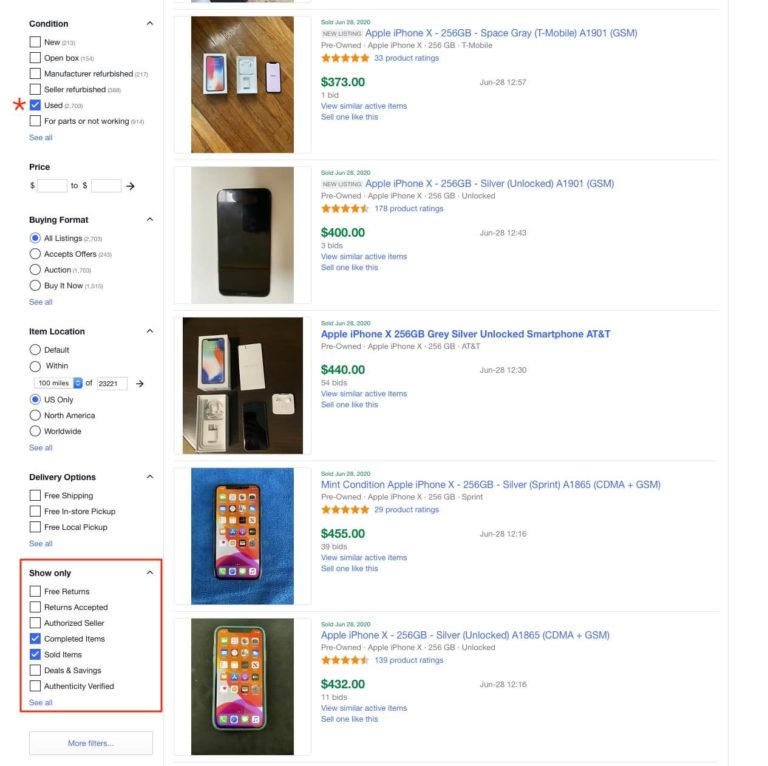In the image, an Amazon webpage is displayed, showing a search for iPhones. On the left-hand side, a filter panel is visible with several options. The user has selected the "Used" condition option, indicated by a checkmark in blue. Below this, the "All Listings" filter is active, marked with a blue dot. Further down, there are options for "Item Location," and at the bottom, there's a section labeled "Show Only," which includes choices for "Completed" and "Sold Items."

On the right side of the page, there are five images of Apple iPhone X models stacked vertically. Each listing includes important details such as price and condition. The first iPhone X at the top is priced at $373. The second iPhone X below that is black and priced at $400. The third iPhone X is listed for $440. Below that, a mint condition iPhone X is priced at $455. The final iPhone X in the series is listed for $432. The prices for these phones are displayed in green text.